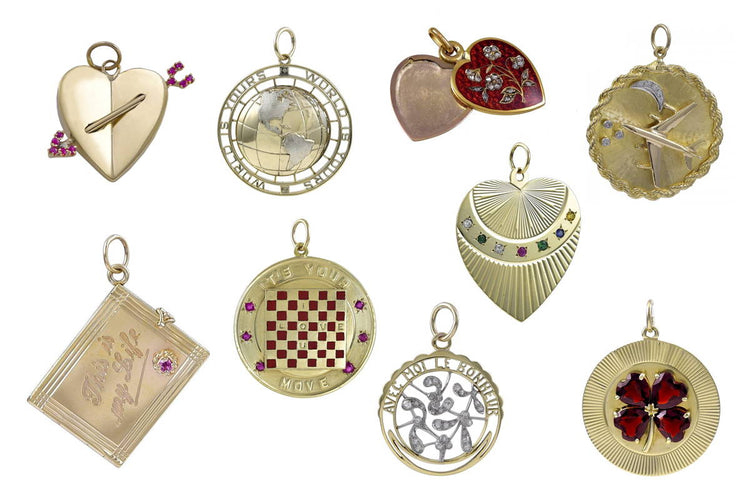The image displays nine intricately designed gold charms, each with a circular hook for attaching to a chain, making them suitable for bracelets or necklaces. The charms are arranged in two rows with four on the top and five on the bottom, set against a white background.

- **Top row**:
    1. A gold heart pierced by an arrow adorned with tiny red stones.
    2. A round medallion featuring a gold and silver globe with the words "The World is Yours" cut out around it.
    3. A heart locket with a red enamel exterior decorated with flowers and a gold bottom.
    4. A round locket with a braided edge, showcasing an inset 3D image of a gold airplane, a crescent moon, and three small diamonds.

- **Bottom row**:
    1. A rectangular charm with a script that reads "This is my life," embellished with a raised flower and a red stone.
    2. A round locket designed as a gold and red checkerboard with the phrase "It's Your Move" circled around it and the words "I love you" interspersed.
    3. A cutout charm with the inscription "Avec moi le bonheur" featuring silver diamond shapes and rhinestones resembling plants.
    4. A four-leaf clover charm made with red stones, set with a small gold piece in the center.
    5. A heart with a curved band adorned with seven multi-colored jewels.

These charms, characterized by their sentimental themes and embellishments with precious stones, seem perfect for gifting on occasions like Valentine's Day. The overall presentation suggests it could be an advertisement for custom-made gold charms and medallions, highlighting their potential as heartfelt gifts that carry deep personal significance.